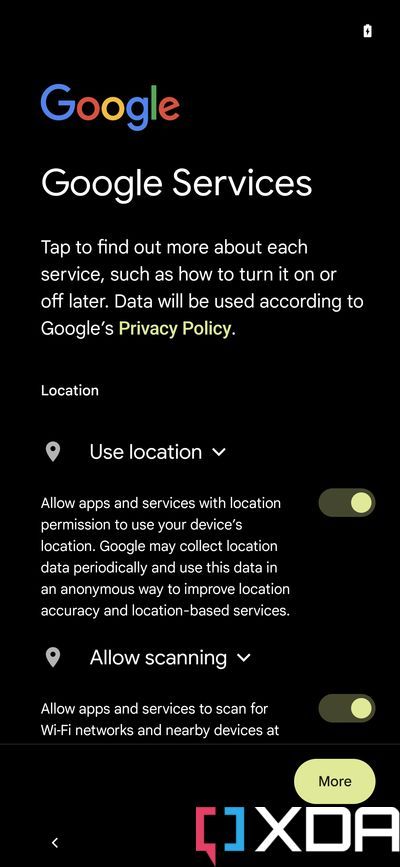The image depicts a dark interface screen containing a detailed set of information regarding Google services and privacy settings. At the very top, the word "Google" appears in a sequence of vibrant colors: blue, red, yellow, blue, green, and red. Below "Google," the text "Google services" is presented in white, centered in a bold, Century Gothic font. 

Beneath this heading, in a slightly smaller and less bold version of the same font, the text reads: "Tap to find out more about each service, such as how to turn it on or off later. Data will be used according to Google's." The phrase "privacy policy" appears next, highlighted in a green font that is slightly bolder than the surrounding text.

Under this, still in white but smaller text, the word "Location" is displayed with an accompanying map pin drop symbol. Next to this, the phrase "Use location" is shown, followed by a downward-pointing arrow, indicating additional information follows. The text explains, "Allow apps and services with location permission to use your device's location. Google may collect location data periodically and use this data in an anonymous way to improve location accuracy in location-based services." This option is toggled on, evident by a light yellow toggle switch with a yellow dot positioned to the right.

Additionally, there is another map pin drop symbol labeled "Allow scanning," followed by a similar downward arrow. The text "Allow apps and services to scan for wifi networks and nearby devices" is partially cut off, but it is clear that this option is also toggled on, indicated by another light yellow toggle switch with a yellow dot on the right.

At the bottom of the interface, there is a rounded, pale yellow oval button with the word "More" written in black. Finally, at the bottom of the screen, the term "QXDA" is displayed, with its 'Q' divided into two colors: dark pink on one side and blue on the other.

This interface image efficiently communicates various settings and permissions associated with Google services, each visually distinct element tailored to ensure clarity and user engagement.